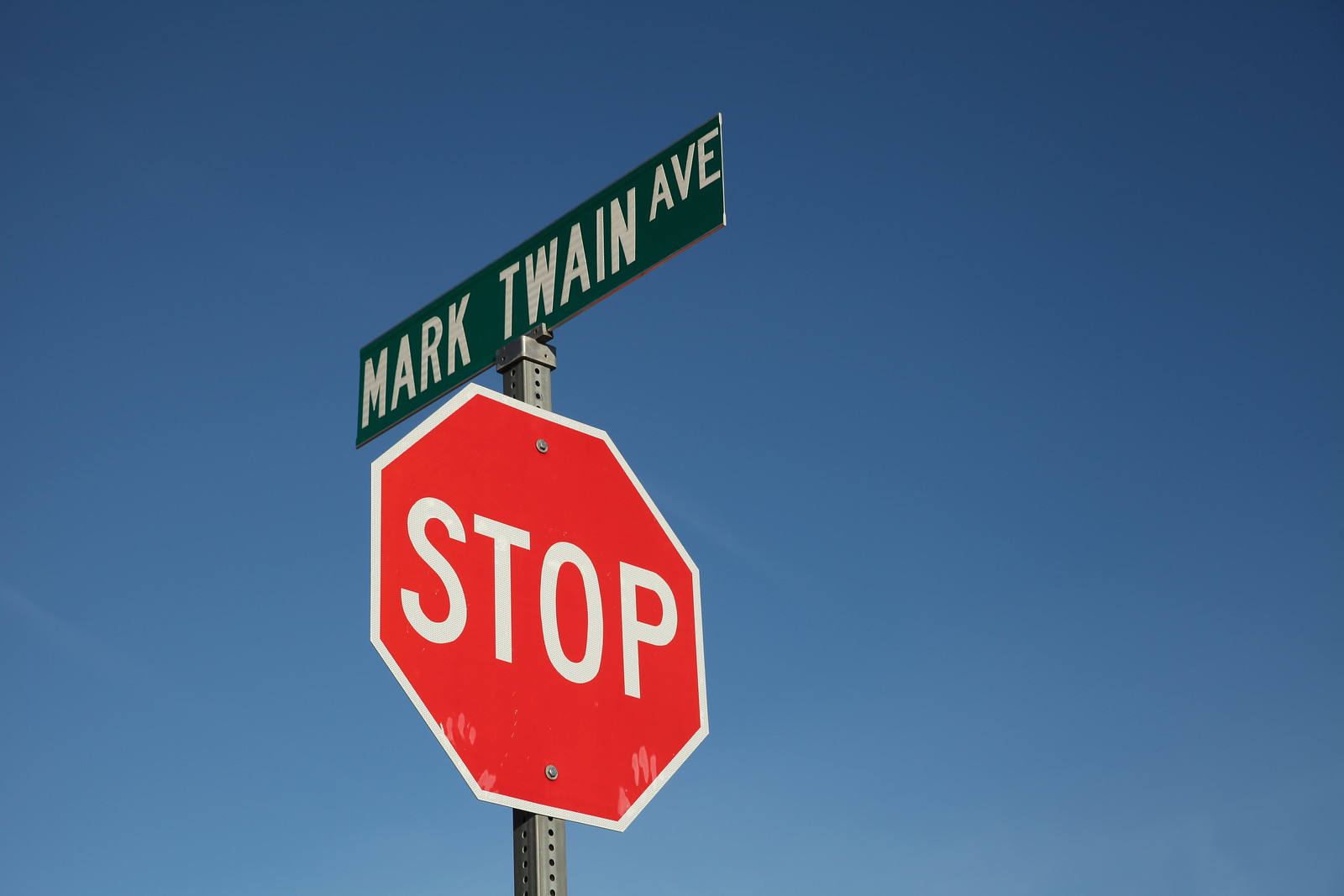The image captures a close-up view of a traditional red stop sign mounted on a square metal pole. The stop sign has a red background, white border, and bold white capital letters spelling "STOP" at its center. Slightly faded and marked by minor spots, the stop sign shows signs of aging and exposure to the sun. Above the stop sign, a green rectangular street sign with white text reads "Mark Twain Ave," indicating the street name. The backdrop of the image is a clear, cloudless blue sky that transitions from a lighter blue at the horizon to a darker blue at the top, highlighting the sunny conditions. The photograph primarily focuses on the upper portion of the metal pole, presenting both the stop sign and the street sign against the vibrant sky.